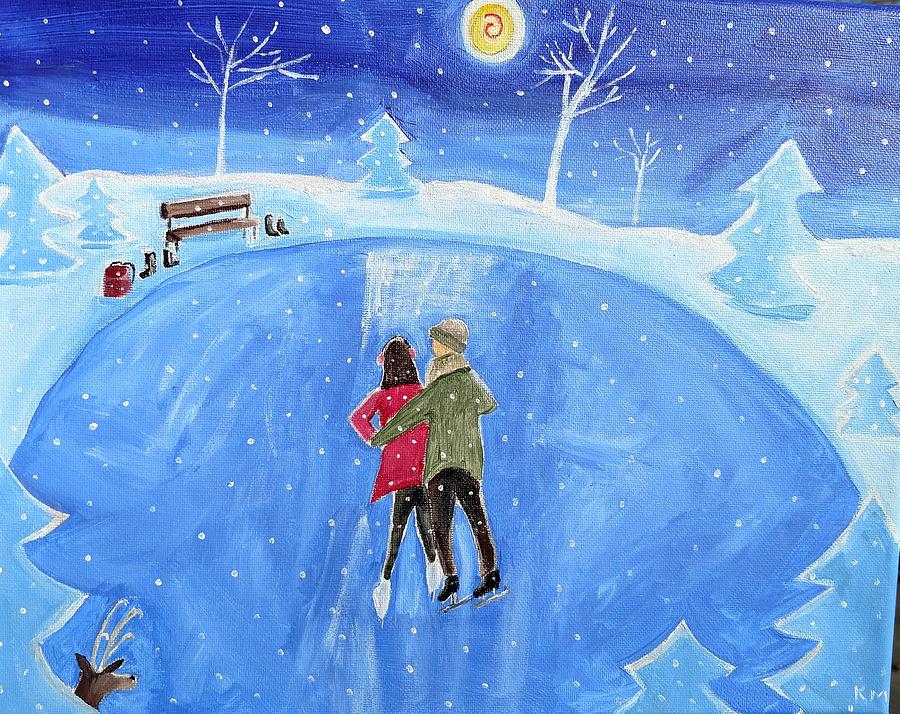This painting on canvas, likely done in acrylic or oil, depicts a serene winter scene rendered in a naive, almost amateurish style. At the center of the image, a pair of ice skaters glide on a frozen blue pond. The female skater, distinguished by her earmuffs, red coat, black pants, and white ice skates, is embraced by her male partner. He wears a brown coat, black ice skates, a knitted brown cap, and black pants. 

Surrounding the pond are classic Christmas-tree shaped pines dusted with snow and other trees with bare branches. A bench sits on the far side of the pond, accompanied by the couple's boots and a red backpack. 

The sky above, painted in a Van Gogh-esque style, features a swirling yellow sun with a red center and is flecked with white snowflakes. In the lower left corner, a deer peeks out from behind one of the pine trees, its curious gaze fixed on the skaters who are unaware of the observer. The artist's initials, K.M., are inscribed in the lower right of the painting, adding a personal touch to this charming winter tableau.